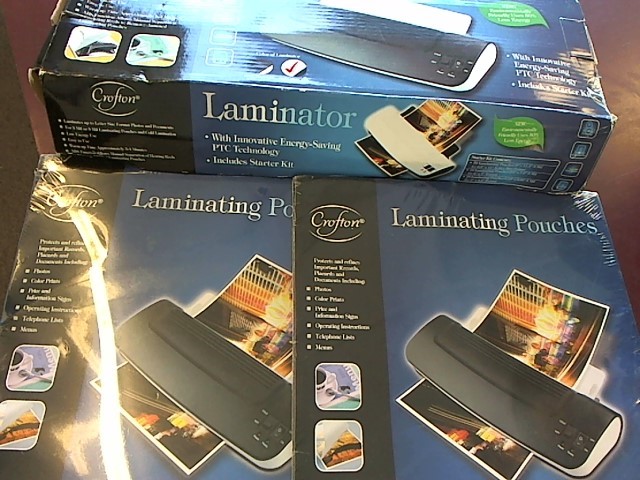The image depicts three blue boxes of CrowFawn laminating pouches, each slightly beat up but still sealed in clear plastic. The topmost box shows only its bottom part, while the middle box is almost fully visible. A prominent black column on each box displays the brand name "CrowFawn" at the top, accompanied by descriptions of the laminating pouches and their features. The boxes feature images of a black laminator machine with a white center, seen processing photos on the left and right sides. Additionally, near the top of the black column, there are pictures of laminated items. Below the brand name, text highlights the product's innovative energy-saving PTC technology. All boxes are situated on a brown floor.